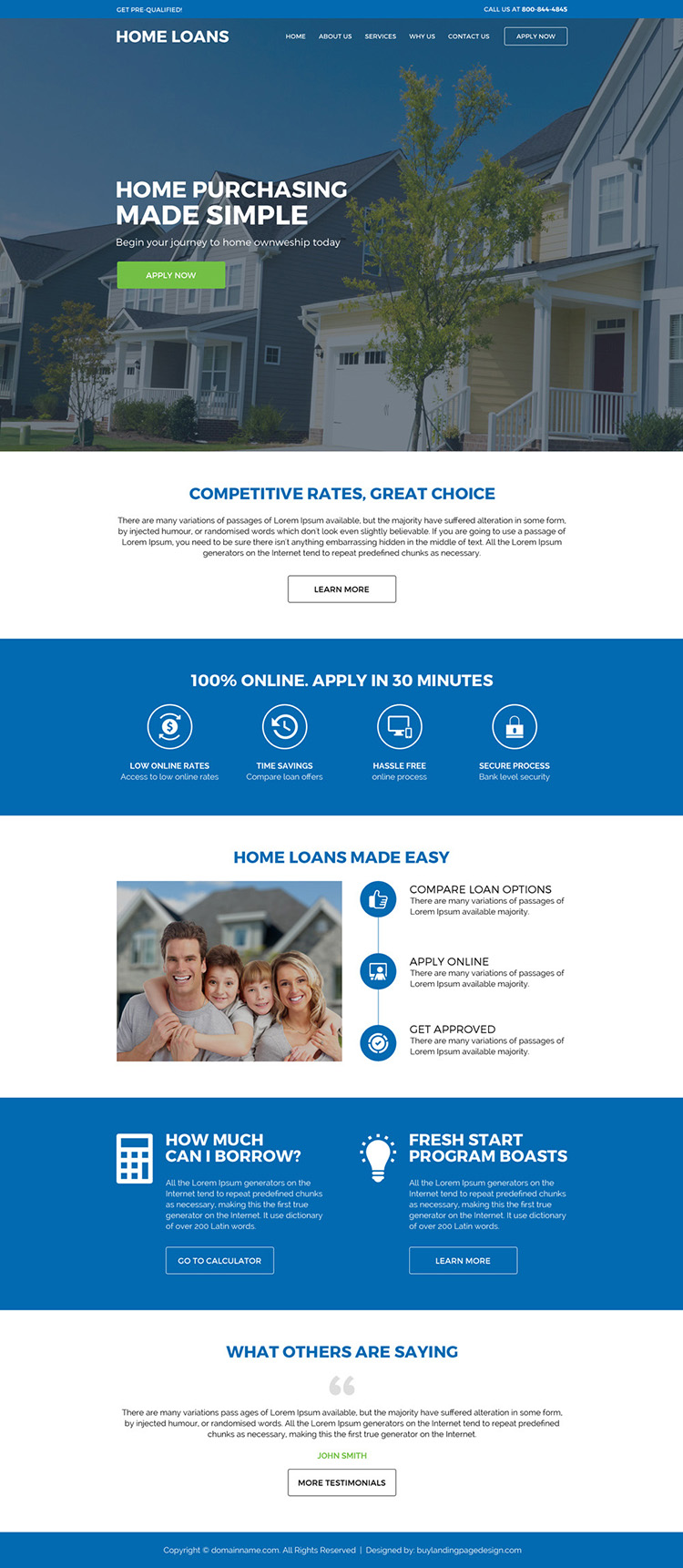The image is a screenshot of a home loan website. At the top, there is a prominent blue banner with the text "Get Pre-Qualified" and a contact number "Call us at 800-844-4845." The banner also features an outdoor scene with a sky, houses, and trees.

Below that, the text "Home Loans" appears, and a horizontal navigation menu is displayed, listing the options: Home, About Us, Services, Why Us, Contact Us, and Apply Now. The menu is outlined with a border.

Further down, a bold heading in all capital letters reads "HOME PURCHASING MADE SIMPLE," with "MADE SIMPLE" in a larger font. Beneath this, there is a call-to-action message: "Begin your journey to homeownership today" accompanied by a green button with "APPLY NOW" written in white.

The next section features a white background and text highlighting competitive rates, great choices, and a "Learn More" option. Adjacent to this is a blue background with key benefits listed: "100% online," "Apply in 30 minutes," "Low online rates," "Time savings," and "Hassle-free and secure process."

Continuing down, a white background holds blue text stating "Home Loans Made Easy," followed by subpoints: "Compare loan options," "Apply online," and "Get approved." An image of a smiling family standing in front of a house complements this section.

The lower part of the webpage contains another blue banner with the questions, "How Much Can I Borrow?" and details about a "Fresh Start Program." Finally, on a white background, there is a section titled "What Others Are Saying" which includes a testimonial, along with a link to read more testimonials.